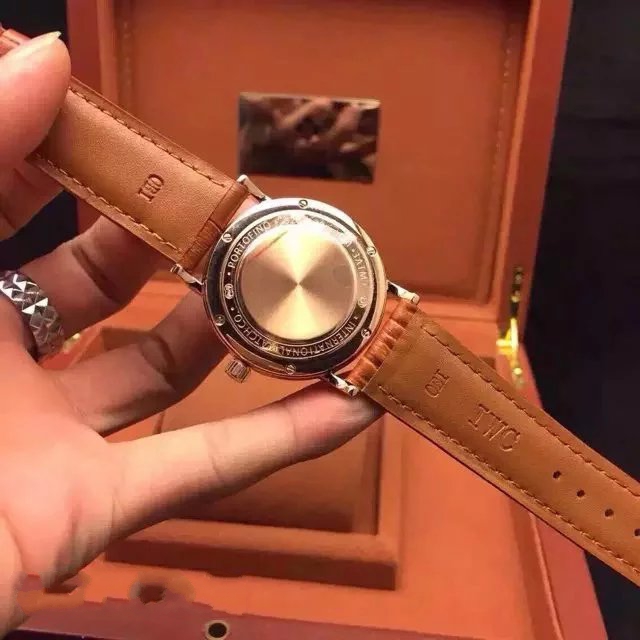This close-up photograph captures the backside of a luxurious wristwatch, bathed in a warm, goldish hue. The watch features a light, warm brown leather wristband, exuding an air of timeless elegance. Held delicately by what appears to be a woman’s hand, as indicated by the slender fingers, well-manicured nails, and a very decorative ring adorning one of her fingers, the watch takes center stage in this image. 

In the backdrop, slightly out of focus, there is a display or protective case, possibly the original packaging of the watch. The case exhibits a brownish, reddish hue, complemented by bright, brassy hinges, which provide a striking contrast to the softer gold color of the watch’s backside. The watch bears inscriptions around its perimeter, reading "Portofino International," though the complete text is partially obscured by a light glare, making the final word difficult to discern. The composition of this photograph underscores the refinement and sophistication of the wristwatch, evoking a sense of luxury and exclusivity.